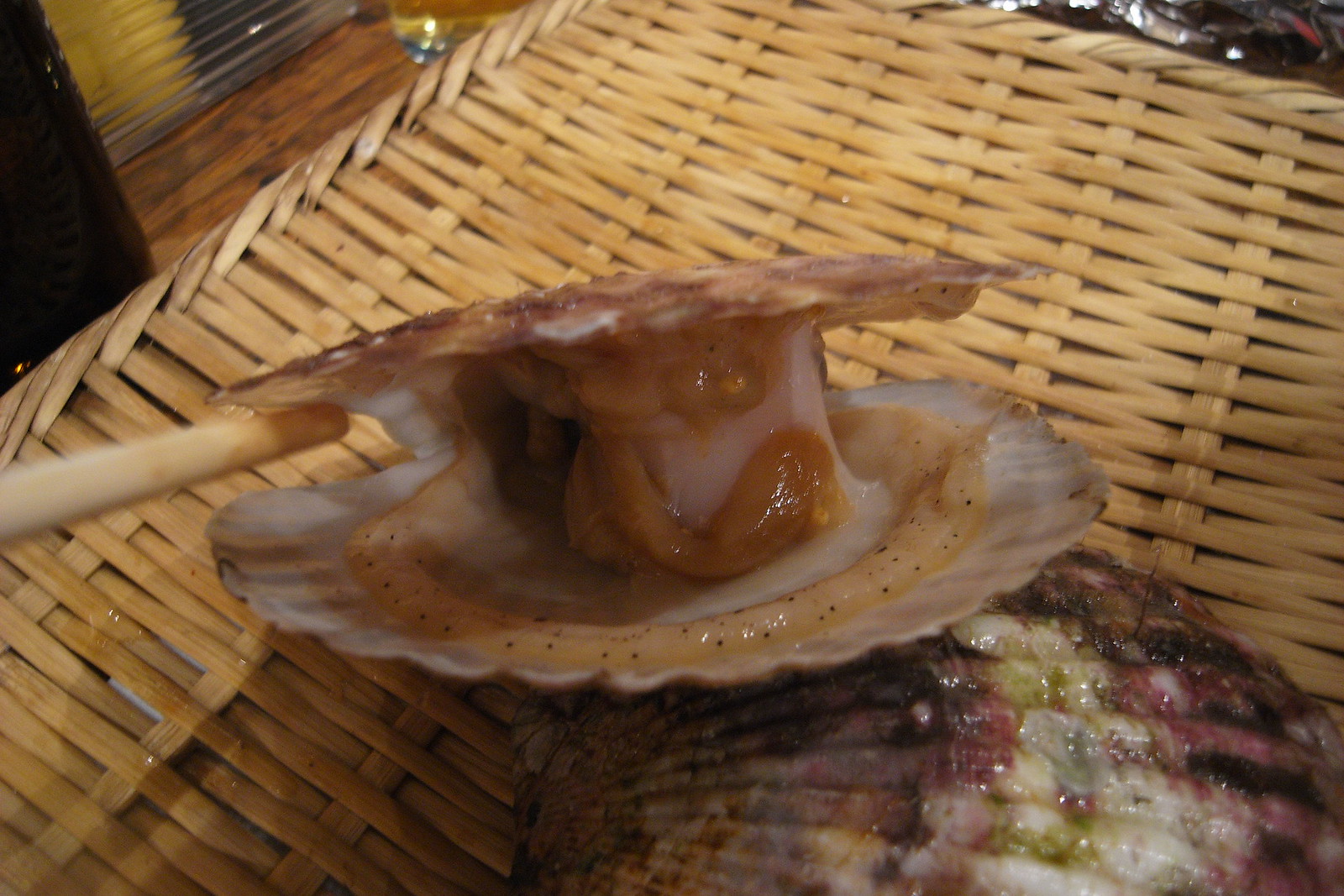The image showcases a detailed culinary display featuring two seashells, resembling clams or oysters. The top shell, pried open by a brown stick, reveals its insides: a slimy, orange and white substance with scattered black dots around the edges. This shell sits atop another similar shell that remains partially open, exposing hints of orange and pinkish interiors. Both seashells rest on a larger, multi-colored seashell – predominantly white with black, purple, and green hues – which creates a striking contrast. The entire arrangement is presented on a wooden, woven basket or platter, set against a textured wooden table. In the background, partially visible objects such as a glass, a plastic ball, and possibly some tinfoil add depth to the setting, suggesting a restaurant environment. A chopstick or similar utensil can be seen on the left side of the image, reinforcing the dining context.